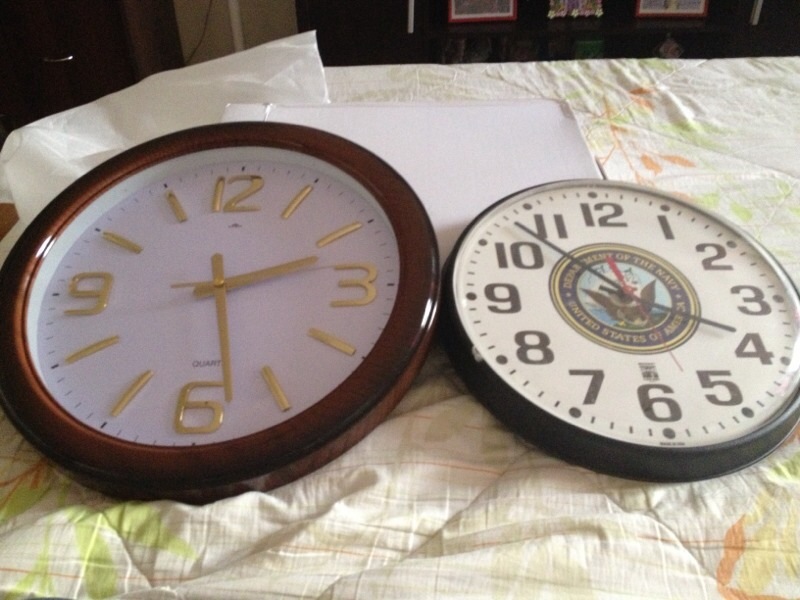Two clocks sit side by side on a gently wrinkled tablecloth that is white with light green and orange patterns. The clock on the left features a possibly wooden, brown frame with a minimalist design: it displays the numbers 12, 3, 6, and 9, with simple lines representing the other hours. Its hour, minute, and second hands are all gold, and it currently shows the time as 2:28. The clock on the right has a black frame and displays all the numbers from 1 to 12. In the center, there is a seal with an eagle, and the text "United States of" is partially visible below it. The time on this clock is 3:53, with black hour and minute hands and a red second hand. Both clocks, circular in shape, provide a striking contrast in their color and design.